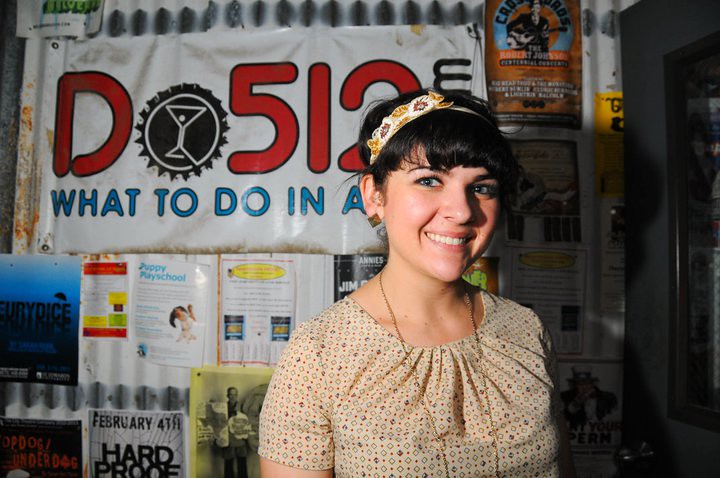In this image, we see a smiling woman, possibly in her late 30s, with short dark brown hair and bangs. She’s wearing a white headband adorned with flowers, as well as gold square or diamond-shaped earrings. Her bright blue eyes are friendly and her teeth are straight and white. She is dressed in a light beige blouse that features various small colored dots or squares, and she has a thin gold chain necklace around her neck. An indistinct banner behind her reads "DO512" in red letters on a white background, and "what to do in a" in blue letters, the rest obscured by her presence. Additional posters and small signs are visible in the background, suggesting a casual venue, possibly a bar, where community events or musical performances are hosted. There’s also a mirror in the far right of the image, reflecting part of her silhouette. The atmosphere feels lively and welcoming, indicative of a social gathering or event setting.